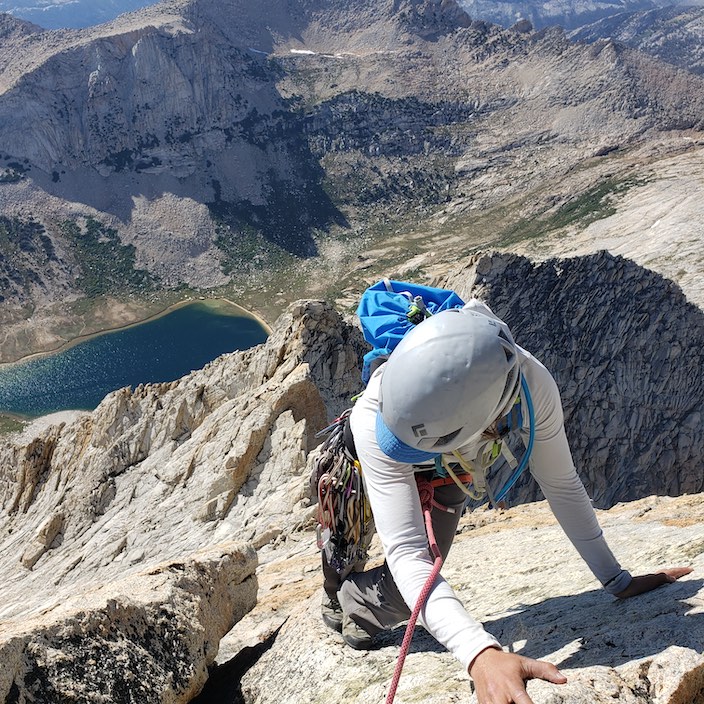This striking outdoor photograph captures a climber, equipped with a red rope, harness, and various climbing gear clipped to their waist, as they near the summit of a towering, rugged mountain. The climber, clad in a white shirt and a gray hat with a blue brim, is seen from above, looking back down over their shoulder, offering a breathtaking view of the expansive landscape below. The scene reveals the climber’s blue backpack and the sheer height of their ascent, emphasized by the tiny, distant features in the background. Bathed in sunlight, a serene lake, surrounded by patches of green grass, glistens at the base of the mountain. The mountain terrain itself is a blend of light limestone brown with intricate shades of gray and veins of black stretching across its surface. Various shadows play across the mountainside, highlighting the stark contrast in its texture. This captivating image not only showcases the climber's daring journey but also the stunning, sunlit beauty of the mountainous landscape.